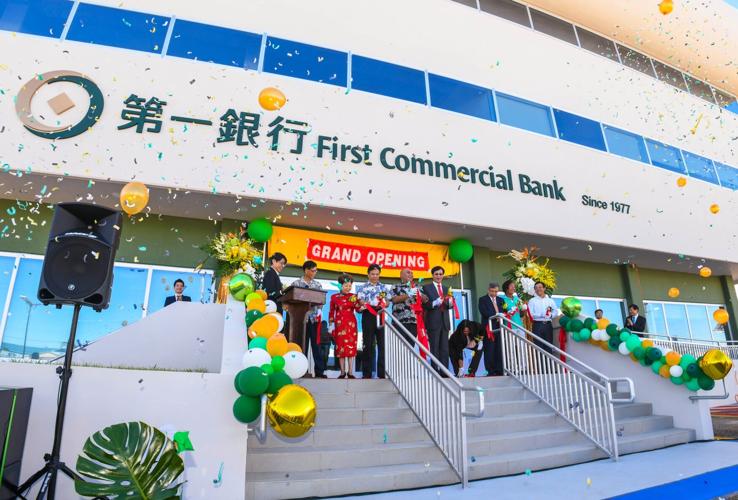This vibrant color photograph captures the front facade of a bank building, prominently displaying the sign "First Commercial Bank since 1977" alongside Asian lettering above its doorway. A central staircase, adorned with banisters, is festooned with an array of colorful balloons in gold, green, white, and orange, adding a festive touch to the scene. To the right of the image, a tall speaker stands on a pedestal, suggesting the presence of an ongoing event or announcement. Cascading confetti falls from the top of the image, enhancing the celebratory atmosphere. In front of a bright yellow and red "Grand Opening" sign, a group of people gathered on the steps appear to be in high spirits, with many clapping and joining in the celebration, marking the joyous occasion of the bank's grand opening.